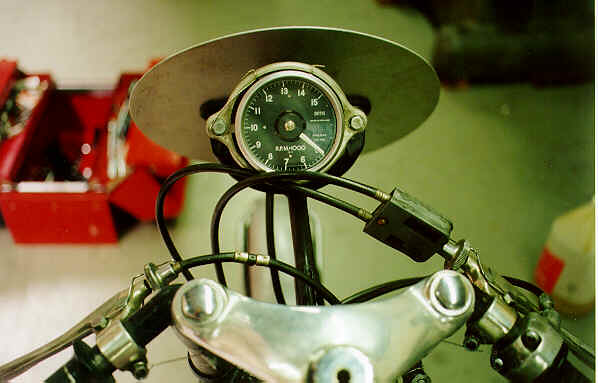The image provides a bird’s-eye view of the front section of a bicycle. Dominating the lower center, a long, curved silver piece features small knobs on either side. The black handlebars are adorned with silver washer pieces and matching silver knobs, which likely serve as screws. Emerging from the upper area, a black wire connects to the silver handlebars, linking to the brake mechanism that cyclists press to stop the bike. Above this, more black wires lead to a small square black box. Notably, a speedometer with a silver encasing is present; its dial, marked from 15 to 5, indicates a reading of five. In the backdrop, an open red toolbox is visible, alongside a large plastic bottle. The bottle is brown with a red label on its front.